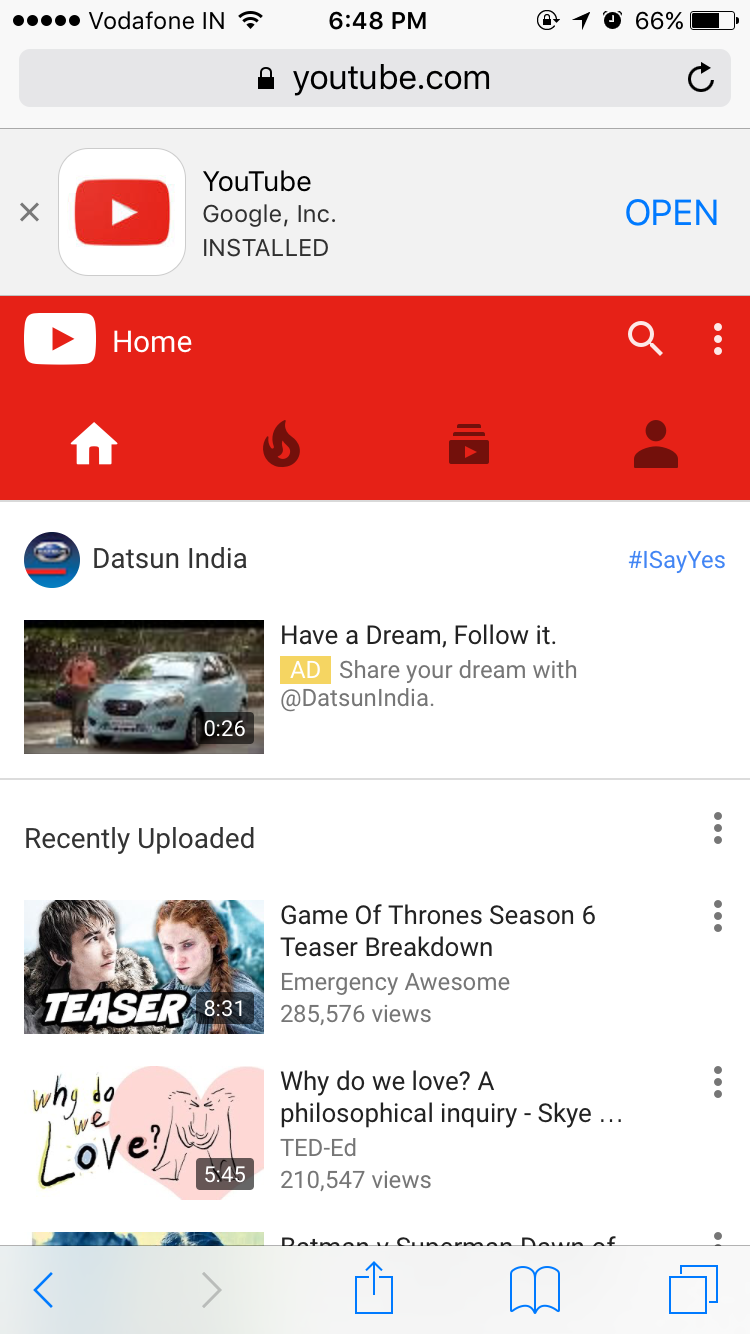A detailed screenshot from a cell phone displays various elements:

- At the top of the screen, there are five dots on a horizontal line followed by the network name "Vodafone I-N" and a Wi-Fi signal icon. The time is centered at 6:48 PM. On the right side, several icons are present, including a battery icon showing 66% charge.

- Below this, a search bar in the center of the screen features a lock icon and the text "YouTube.com." To the far right of the search bar is a circular arrow icon.

- Beneath the search bar, there is an 'X' symbol next to the YouTube logo, followed by the text "YouTube Google Inc installed" and a button labelled "Open" in blue text on the right.

- Further down, a red bar is visible with the YouTube icon. "Home" is displayed in the upper left corner of the bar, while a magnifying glass icon and three vertically stacked dots are on the upper right.

- Under this bar, four icons are displayed horizontally: a white home icon, a gray fire icon, a gray file icon, and a gray person icon.

- Continuing below, YouTube entries appear:

    - The first entry starts with "Dotson India" on the upper left and "#I say yes" on the upper right of the box. It features an image of a car and a woman standing beside it, dressed in a pink shirt, brown pants, and carrying a black bag. It carries the text: "Have a dream, follow it, share your dream with Dotson India."
    
    - The next entry below it is for the "Game of Thrones Season 6 Teaser Breakdown" featuring a picture of a man and woman. The teaser timestamp "8:31" is shown in the lower right corner.

    - Another YouTube entry follows, containing an image of a heart and the text "Why Do We Love." In the lower right of the image, it says "5:48." To the right, the details are "Why Do We Love-A Psychological Inquiry, TED" with 2,547 views.

- At the bottom, a gray bar with multiple icons appears. These include, from left to right: a left-pointing arrow, a right-pointing arrow, an upward-pointing arrow inside a box, a foot icon, and two overlapping squares in the lower right corner.